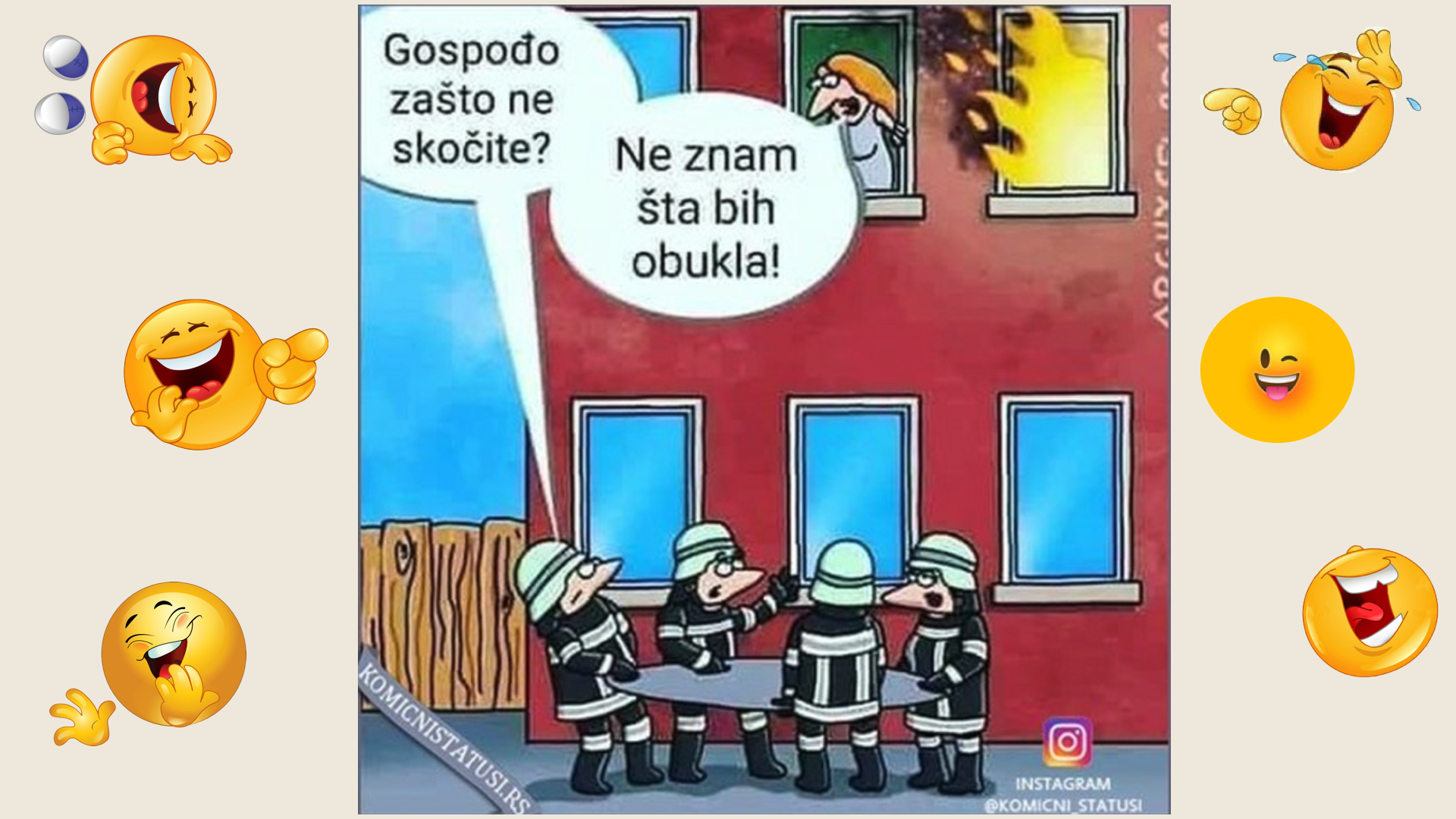This image is a humorous cartoon comic set in a red apartment building with vivid details. A woman, standing in the middle window on the second floor, looks down at four firemen, who are holding a circular jump net at the bottom. Flames are bursting out of the window to her right, indicating a fire emergency. Despite the dire situation, the scene is filled with comedic undertones, emphasized by numerous laughing emojis—three on the left and three on the right side of the comic. The firemen and the woman have speech bubbles written in an unknown language, adding to the comic's mystique. The building features blue windows, except for the one ablaze, and there is a small fence to the left of the building. The firemen are depicted in full gear, including helmets and firecoats. The bottom right corner of the image displays the Instagram logo along with the handle "K-O-M-I-C-N-I underscore status I," indicating its source. The overall presentation suggests that the cartoon is intended to be light-hearted and amusing despite the chaotic scenario it depicts.